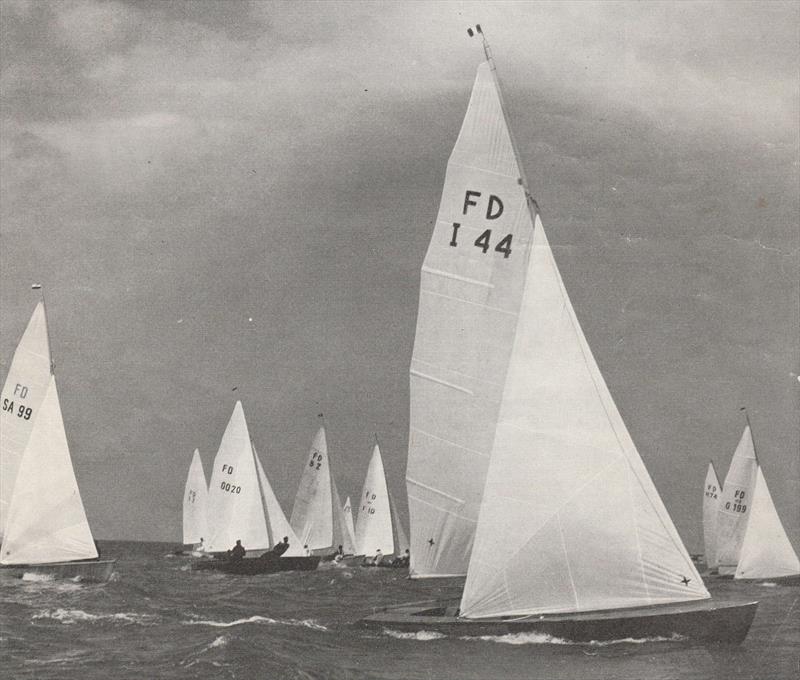This black-and-white photograph captures an intense sailing race on a rough, gray ocean dotted with white caps. The image showcases a fleet of nearly identical sailboats, each with two white, triangular sails marked with distinctive identification numbers such as FDI 44, FOGO 20, and FDSA 99. The shot focuses on one sailboat in the foreground, distinguished by its black-gray hull and the inscription "FDI 44." Sailors, appearing as silhouettes, can be seen maneuvering these boats amidst the choppy waters. The scene is framed by a cloudy, overcast sky, adding to the dramatic atmosphere of the racing event. The image effectively conveys the excitement and chilly ambiance of this competitive sailing race.